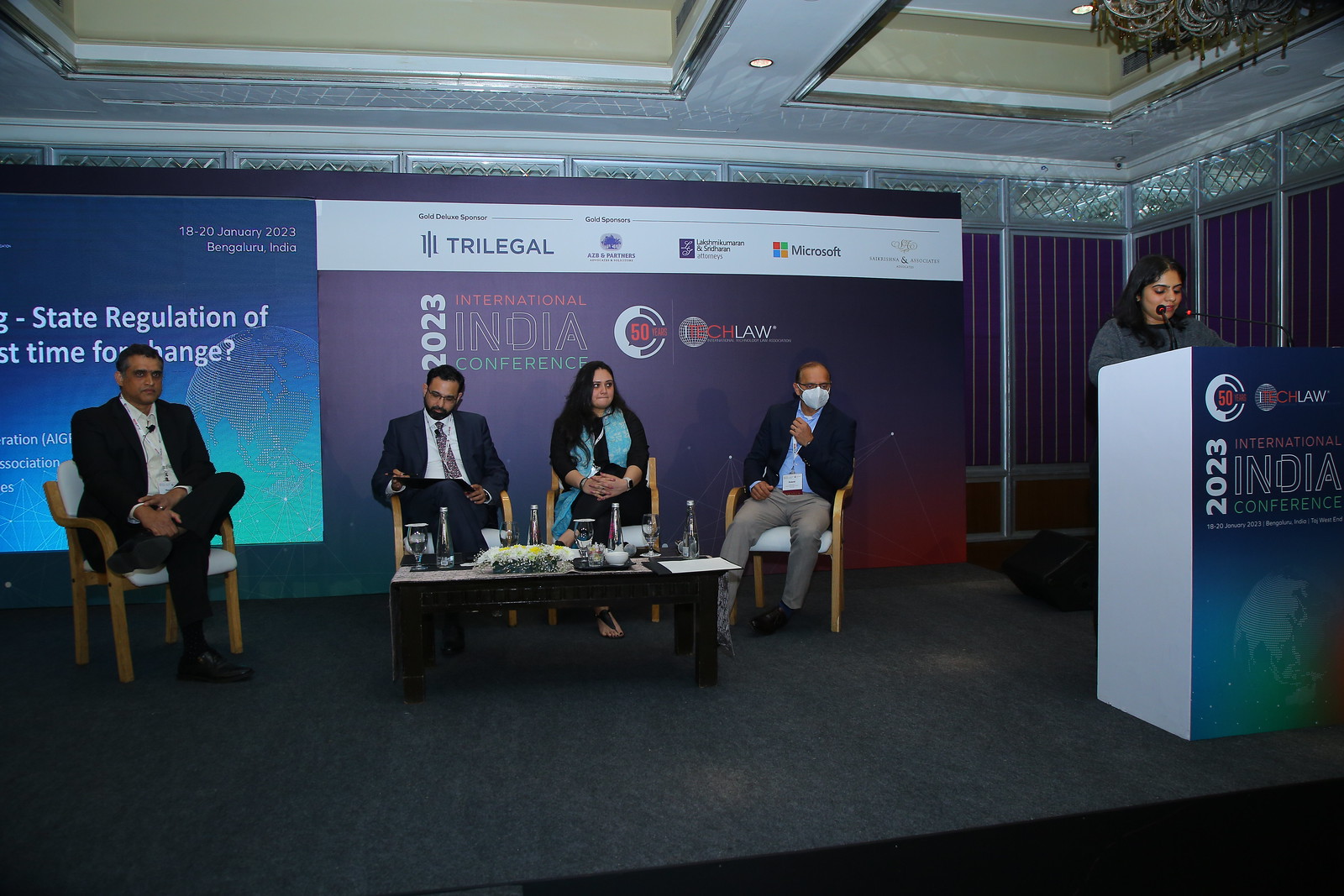The image captures a moment from the 2023 International India Conference. On the right side of the stage, an Indian woman with black hair is speaking energetically at a podium bearing the event's name. She wears a gray shirt and stands behind a microphone. To her immediate left, four Indian attendees sit in brown chairs, attentively listening. The first gentleman on the right wears khaki pants, a blue shirt, a black blazer, and a white mask, with a visible name tag. Beside him, a woman with long hair dons a black jacket, blue shirt, and black pants. Next to her, another man in a suit, with glasses, a beard, and a mustache, examines a document intently. The final person, a man in a black suit with a white shirt, has his legs crossed. A small table is situated in front of them. The backdrop features a large screen and a banner displaying "2023 International India Conference" along with sponsor logos, including Microsoft. The stage itself is gray and elevated, with silver window panels behind it. The ceiling above has two square cut-outs, adding a modern architectural touch to the venue.